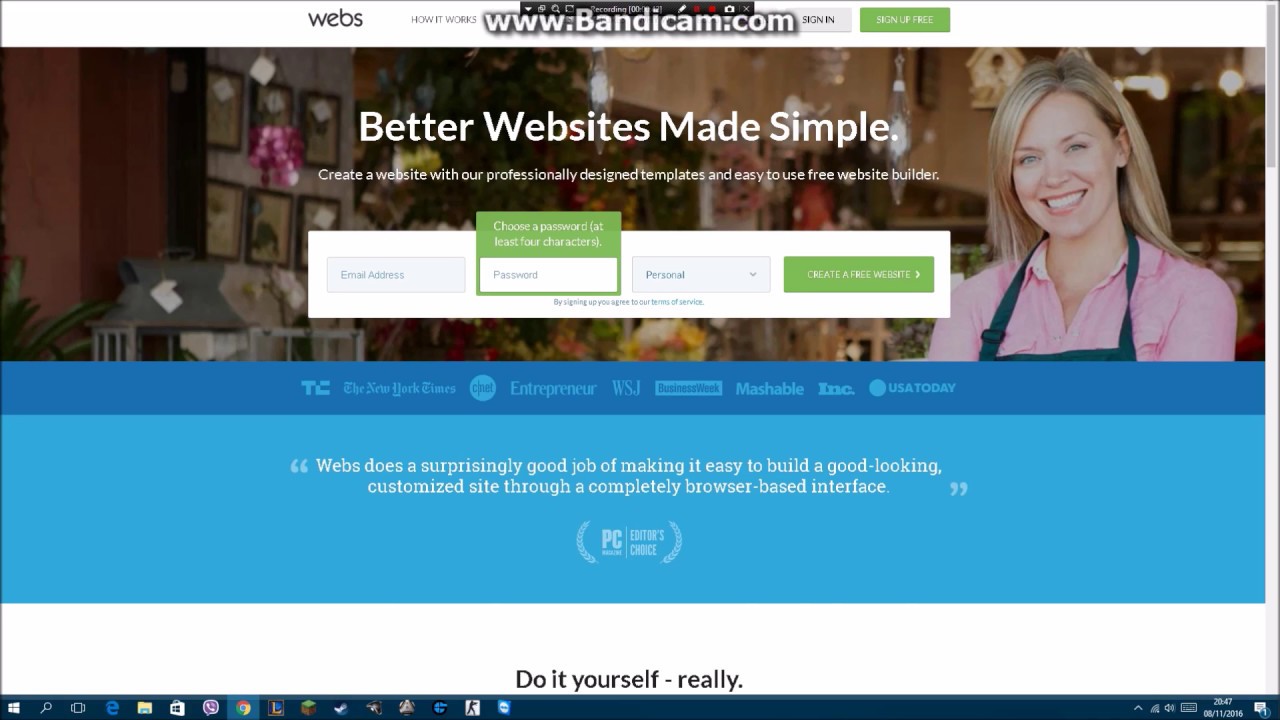The image is a screenshot of a webpage, displayed in landscape mode. At the top center, there is a small black mark indicating that a screen recording is in progress, accompanied by a watermark at the bottom that reads "www.bandicam.com." 

The upper portion of the webpage features a white stripe running from the upper left to the upper right corner, displaying the text "WEBS" and beneath it, the phrase "How it Works." To the right of this stripe are two buttons: a light gray "Sign In" button and a green "Sign Up Free" button.

The background of the webpage depicts what appears to be an indoor retail space, filled with various items for sale, complete with price tags. On the right side of the image, there is a light-skinned woman with blonde hair, wearing a pink shirt and an apron. 

Centrally positioned on the page is the text "Better websites made simple," followed by a description: "Create a website with our professionally designed templates and easy-to-use free website builder."

Below this text is a white form for user registration. The form fields include "Email address," a green background field labeled "Choose a password" along with the instruction "At least four characters," a "Password" field, and a drop-down menu labeled "Personal." At the bottom of the form, there is a green button that reads "Create a free website," accompanied by a disclaimer stating, "By signing up, you agree to our Terms of Service." At the very bottom of the image, it reads, "Do it yourself."

This comprehensive descriptive caption delivers a detailed overview of the webpage's elements, visuals, and textual content.